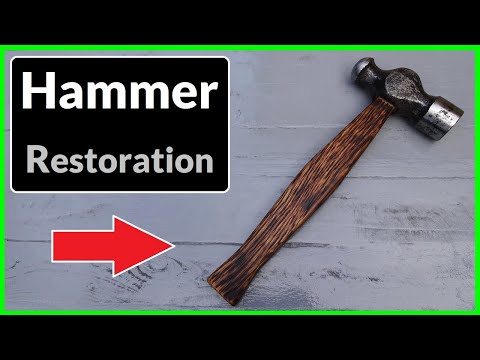The image is a detailed photographic advertisement for hammer restoration, featuring a prominently displayed hammer with a worn, dark wooden handle and a weathered black and silver metal head. The hammer rests diagonally from the bottom left to the top right on a grey whitewashed wooden platform, set against a predominantly black background. The upper left corner of the image contains a black rectangular box, with the word "Hammer" written in white and "Restoration" in grey, matching the grey tones of the wooden background. A solid red arrow outlined in white points towards the hammer, drawing attention to it. Encasing the main part of the image is a neon green border, creating a striking contrast against the black borders at the top and bottom of the picture.